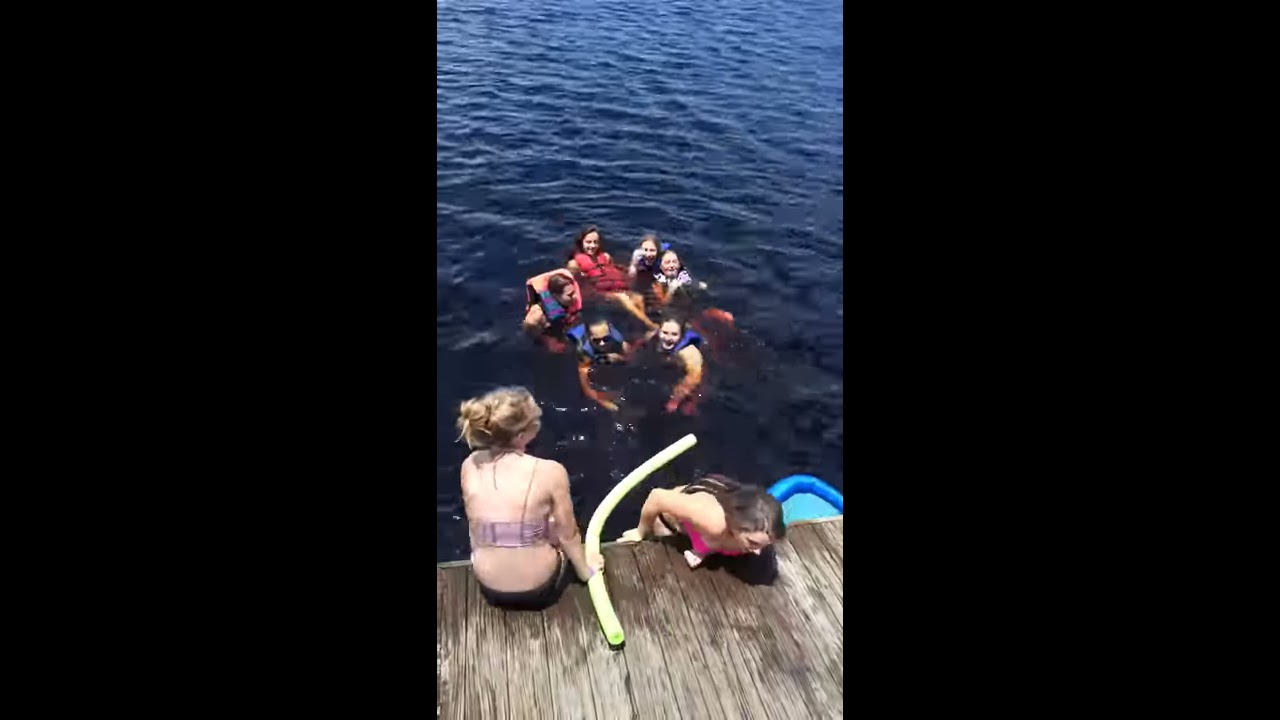The image depicts a wooden dock with eight people near and around it. On the left side of the dock, a woman with light brown, almost blonde hair tied up is sitting, wearing a purple bikini top and black swimsuit bottoms. She is holding a yellow flotation device in her hand. Next to her, a woman with long, dark brown hair cascading down her back is climbing up onto the dock. This woman is wearing a pink bikini top and brown bottoms and appears halfway onto the dock, with her stomach pressed against its edge and her nose facing down towards the wood. 

In the water beside the dock, six individuals wearing life vests are grouped together. Among them, three are in blue life vests at the front, while the other three in the back have two in blue life vests and one in a red life vest. The group in the water forms a circle with their bodies close to each other. The water around them is a dark blue with ripples, but in the upper portion of the image, it turns a lighter blue and appears slightly wavy. Below the woman climbing the dock, a small corner of a light blue object is visible floating in the water. The wooden dock looks aged and dry except where it has been wet by the individuals' bodies. A tip of a blue boat can be seen near the bottom right, partly obscured under the dock. The entire image is framed by broad black borders on the left and right sides.